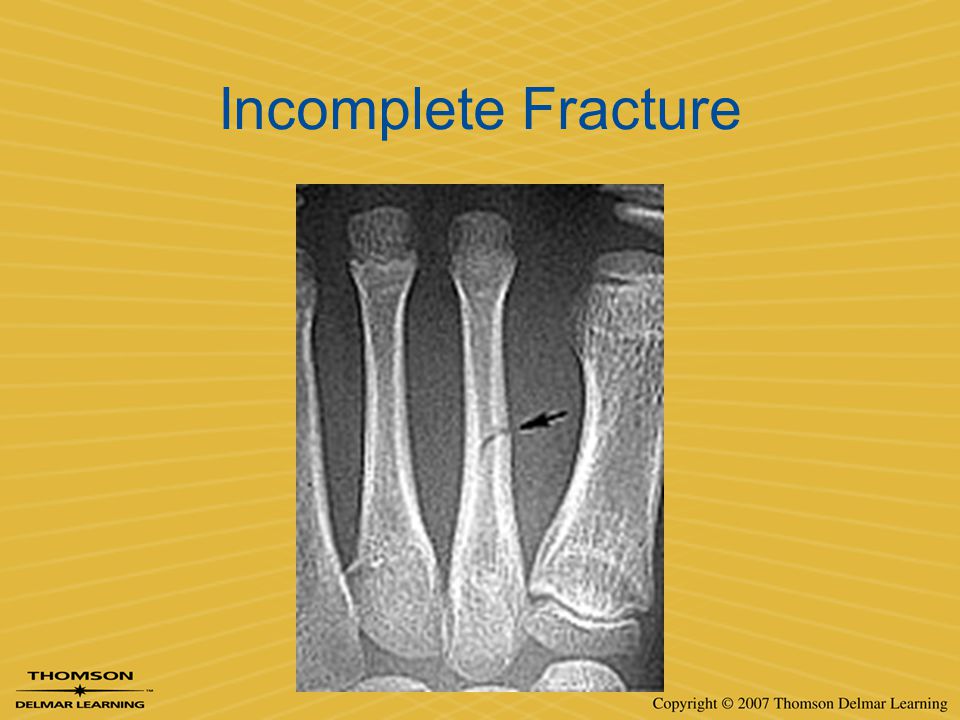The image features an informational slide, likely intended for a medical presentation, set against a mustard yellow to goldenrod background with faint, non-horizontal white lines creating a subtle hatch pattern. Prominently centered at the top, the headline "Incomplete Fracture" is written in a dark blue, sans-serif font with capitalized initial letters. Below this title, a vertical black-and-white radiograph displays four closely aligned bones, likely fingers or toes. The thickest bone on the right bears a fracture, highlighted by a black arrow pointing towards it. At the bottom left corner, the logo reads "THOMPSON" in all caps, followed by a horizontal line with a star, and beneath it, "Del Mar Learning" in smaller uppercase letters. The bottom right corner contains the text "Copyright © 2007 Thompson Delmar Learning" in small black font.